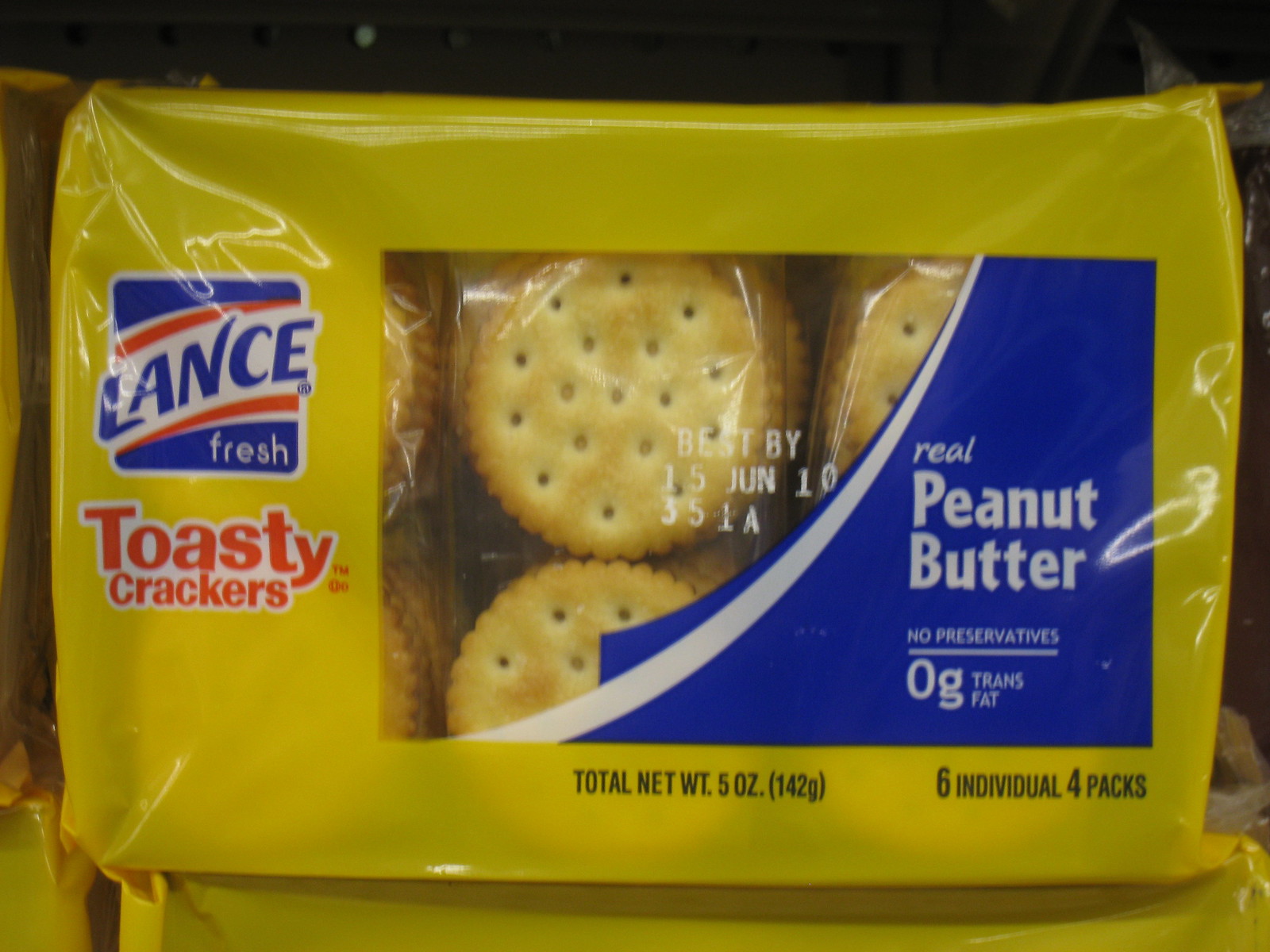This image shows a yellow plastic package of Lance brand Toasty Crackers with peanut butter filling. The packaging features a blue square on the top left with "Lance" written in white text. Below it, the word "fresh" appears. In large red letters at the bottom of the left section, it states "Toasty Crackers." A clear window in the center reveals the circular cracker sandwiches, with visible peanut butter filling through small holes. To the right, a blue section displays the text "real peanut butter," along with "no preservatives" and "zero grams trans fat." The package indicates a "Best by 15 June 10" date and provides nutritional information at the bottom, stating "Total Net Weight 5 ounces (142 grams)" and "6 individual 4 packs."